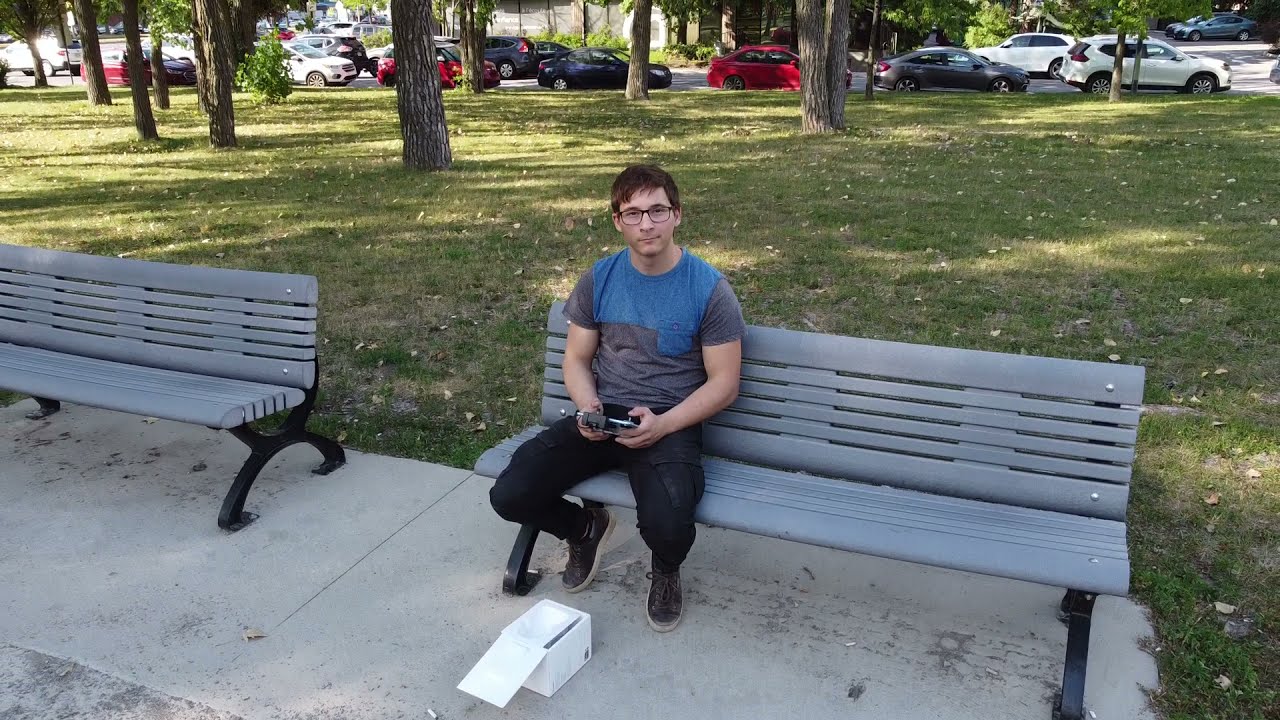The photograph captures a young man with brown hair and dark-rimmed glasses sitting on a gray park bench with black legs. He is dressed in a blue and gray short-sleeve shirt, black pants, and black sneakers. In his hand, he holds a gadget, which he appears to have taken out from an open white box on the light gray concrete sidewalk at his feet. The scene is set in a park, with green grass dotted with small white flowers and several upright brown tree trunks visible behind him. The greenery extends to about 90% of the image before giving way to a street lined with parked cars, including white, black, and red vehicles, as well as a bus. Another identical gray bench sits next to him on the diagonal. The young man has a slight smirk on his face, suggesting he is either using or examining the gadget he has just unboxed.